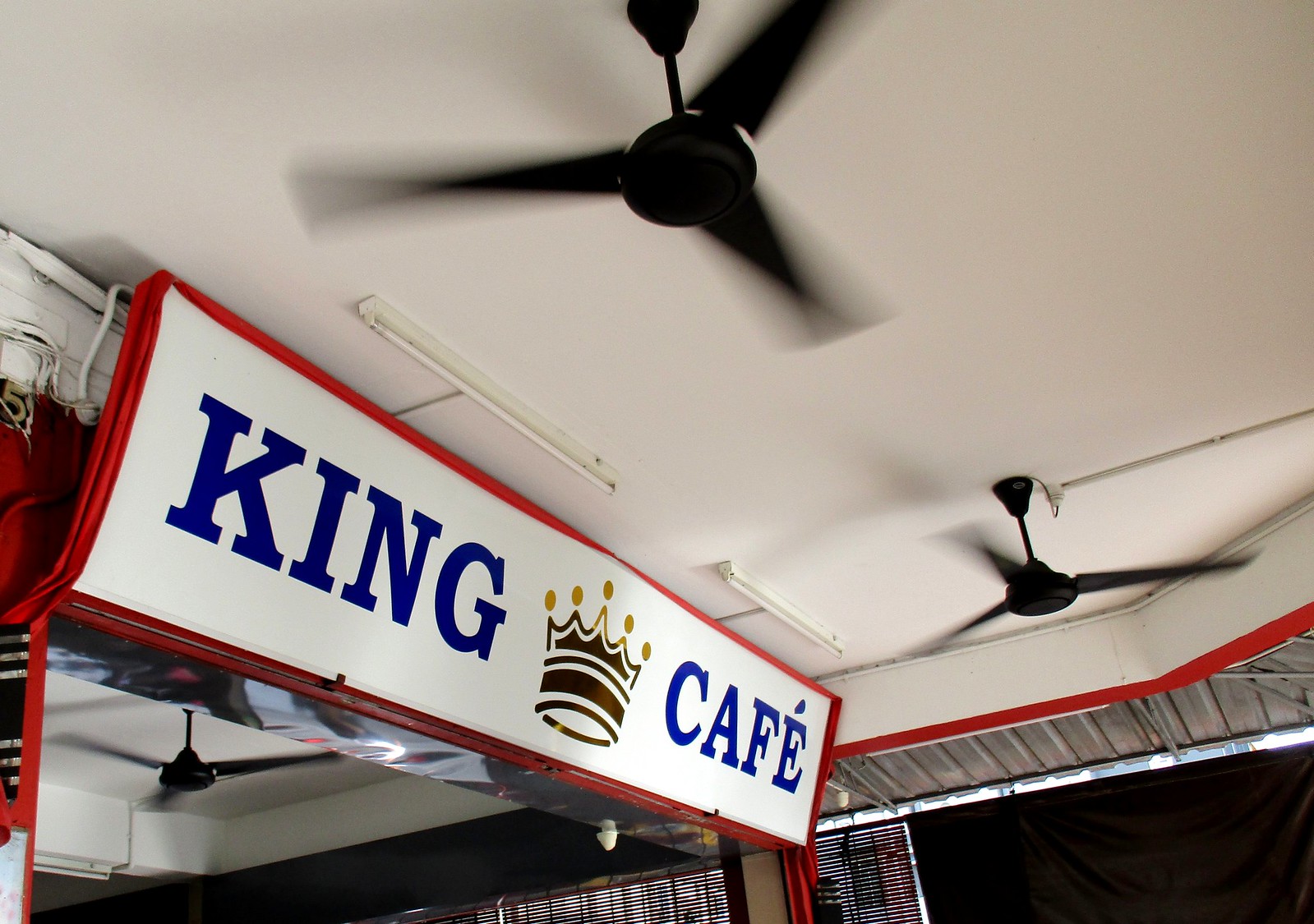In this low-angle shot, we see the white ceiling of what appears to be an open-air restaurant or café. Prominently featured on the ceiling are two black ceiling fans, each with three blades, spinning gently. To the left side of the image, mounted near the top of the wall, is a large white sign bordered in red. The sign displays the words "King Cafe" in big blue letters, with a gold and brown crown illustration positioned centrally between the two words. Also visible are some black curtains and window blinds, suggesting the café may be open to the outside air, with curtains serving to mitigate the elements. A red border can be seen around the ducting on the far right side of the wall, further detailing this inviting and relaxed café environment.